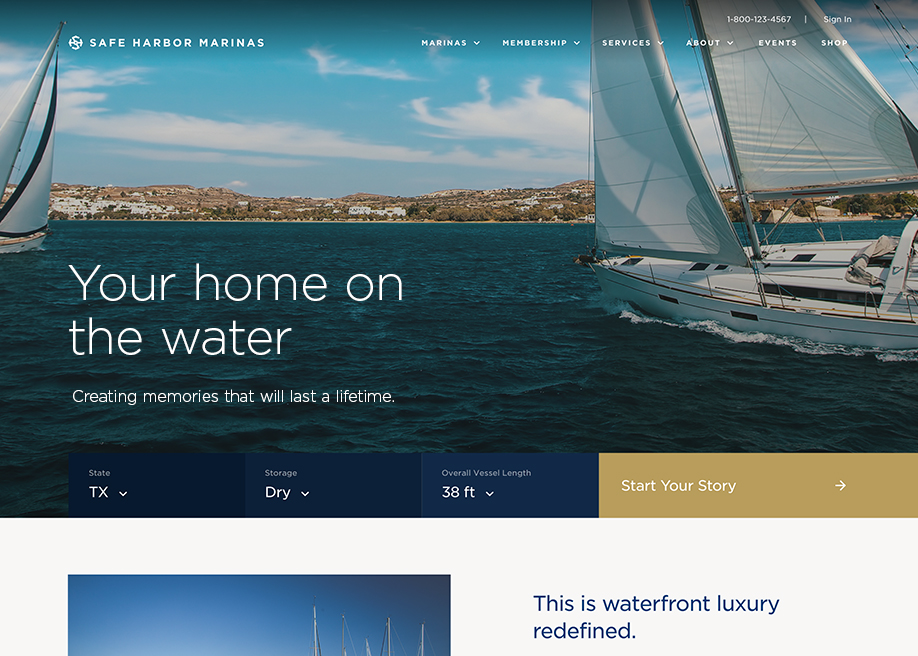A picturesque view from the water showcases two sailboats, predominantly white, positioned on opposite sides of the frame. The expansive dark blue water stretches between them, leading to a distant, low-lying land and a vast blue sky speckled with clouds.

In the upper left corner of the image, text reads "Safe Harbor Marinas." To the right, starting from the middle, are navigation options for "Marinas," "Membership," "Services," "About," and "Event Shop," each accompanied by a drop-down arrow. Above these, the contact number "1-800-123-4567" and a "Sign In" option are visible.

In the lower left portion of the image, text warmly invites viewers with "Your home on the water, creating memories that will last a lifetime." Directly below this, a selection strip features "State: Texas" with a drop-down, "Storage: Dry" with a drop-down, "Overall Vessel Length: 38 feet" with a drop-down, and a prompt to "Start Your Story" with a right arrow.

Below this strip, a partially visible photograph of sailboat masts peeks in, with text proclaiming, "Waterfront luxury redefined" in blue on a white background. This white background begins below the drop-down areas, transitioning the overall scene from the vibrant colors of blue, gold, white, and brown to a clean, white space as it descends.